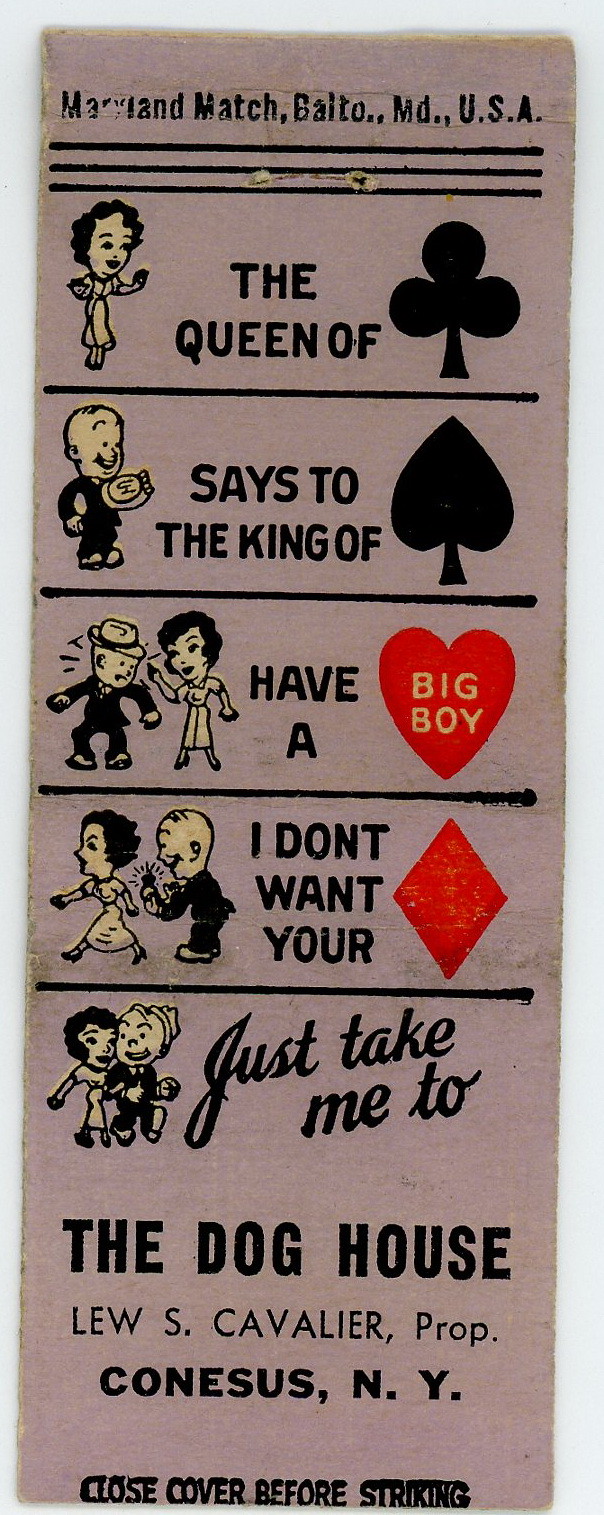This is an image of an old advertisement, possibly a magazine cutout, set against a light purple background. The narrow piece of paper features cartoon figures divided into sections. At the top, it reads "Maryland Match, Baltimore, Maryland, USA" with black divider lines beneath. Below, a drawing of a woman is captioned "The Queen of Spades." Next, a bald man is depicted with the caption "To the King of Spades." Further down, an illustration shows a man and a woman arguing, accompanied by the text "Have a heart, big boy," with a red heart shape nearby. In the following section, another scene shows a man proposing to a woman walking away, under the caption "I don't want your diamond," with a red diamond symbol. The final section reads "Just take me to The Doghouse," mentioning "Lou S. Cavalier, P.R.O.P., Kinesis, New York," followed by the instruction "Close cover before striking."